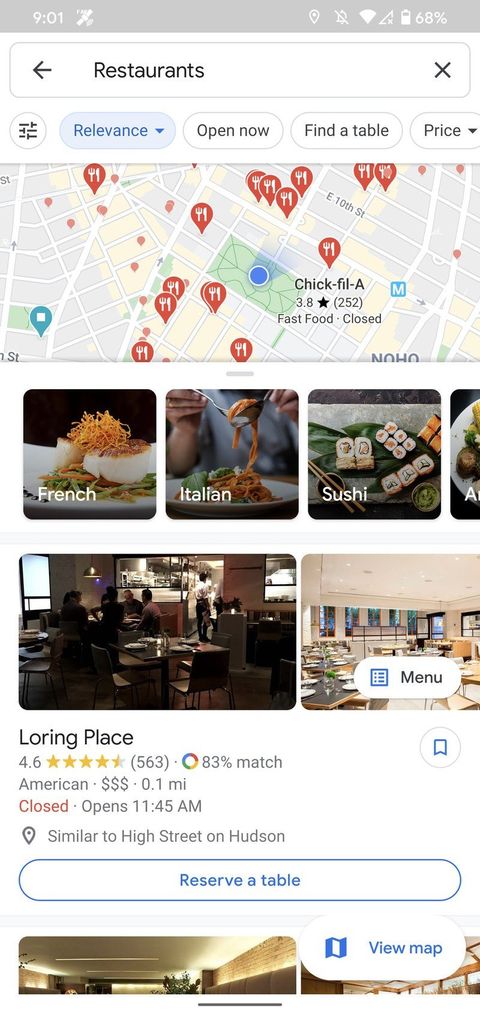### Detailed Caption for Image

This image is a cell phone screenshot showcasing the Google Maps interface on a device running iOS. The user has navigated to the Google Maps search page, specifically looking for nearby restaurants. 

#### Top Section:
At the very top, the phone's notification bar is displayed with typical status indicators: the current time (9:01), and icons showing the phone's data and Wi-Fi signal strength along with the battery life, which is at 68%.

#### Search Bar:
Just below the notification bar, the search bar is featured prominently. The user has typed the term "restaurants" in black text, indicating their search for dining options in the vicinity.

#### Map View:
Directly beneath the search bar is a dynamic map. A blue dot on this map marks the user's current location, surrounded by numerous red dots that signify various restaurants in the area. 

#### Cuisine Options:
Further down are visual icons representing different types of cuisine categories like "French," "Italian," and "Sushi." Each category is depicted with an image related to the type of cuisine it represents—for example, the "Sushi" category displays a picture of sushi dishes. Selecting any of these categories provides more details about the respective type of restaurants.

#### Featured Restaurant:
The bottom half of the page highlights a specific restaurant named "Loring Place." This section includes images, videos, and detailed information such as the restaurant's address, hours of operation, and customer reviews from Google. Reviews and other interactive links offer further insights into the dining experience at "Loring Place."

This detailed caption provides a thorough overview of the features and information visible in the screenshot, making it clear for users unfamiliar with the original image.